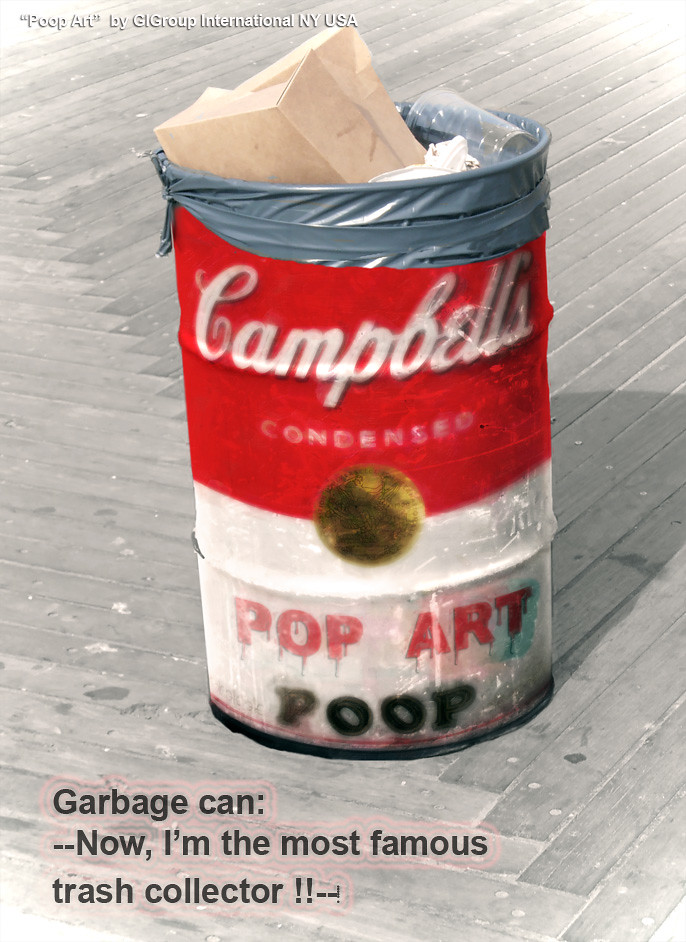This photograph features a cylindrical metal trash can, meticulously painted to resemble a Campbell's condensed soup can in a parody of Warhol’s iconic pop art. The top half of the trash can is red, adorned with the classic white "Campbell's" lettering and a smaller white font that reads "condensed" beneath it. A gold circular medallion is prominently displayed below these texts, dividing the red top from the white lower half of the can. Below the medallion, the words "pop art" appear in red, followed by "poop" in bold black capital letters.

The trash can is placed on a flat wooden surface comprised of light grayish planks, which intersect diagonally, creating a distinctive background pattern. Adding to its artistic nature, the trash can holds a gray industrial trash bag, inside of which are various trash items like cardboard boxes and plastic cups. At the top of the photograph, a watermark reads "poop art by G.I. Group International, New York, USA." Complementing this, a text overlay in the lower-left corner announces, “garbage can: --now, I’m the most famous trash collector!!”